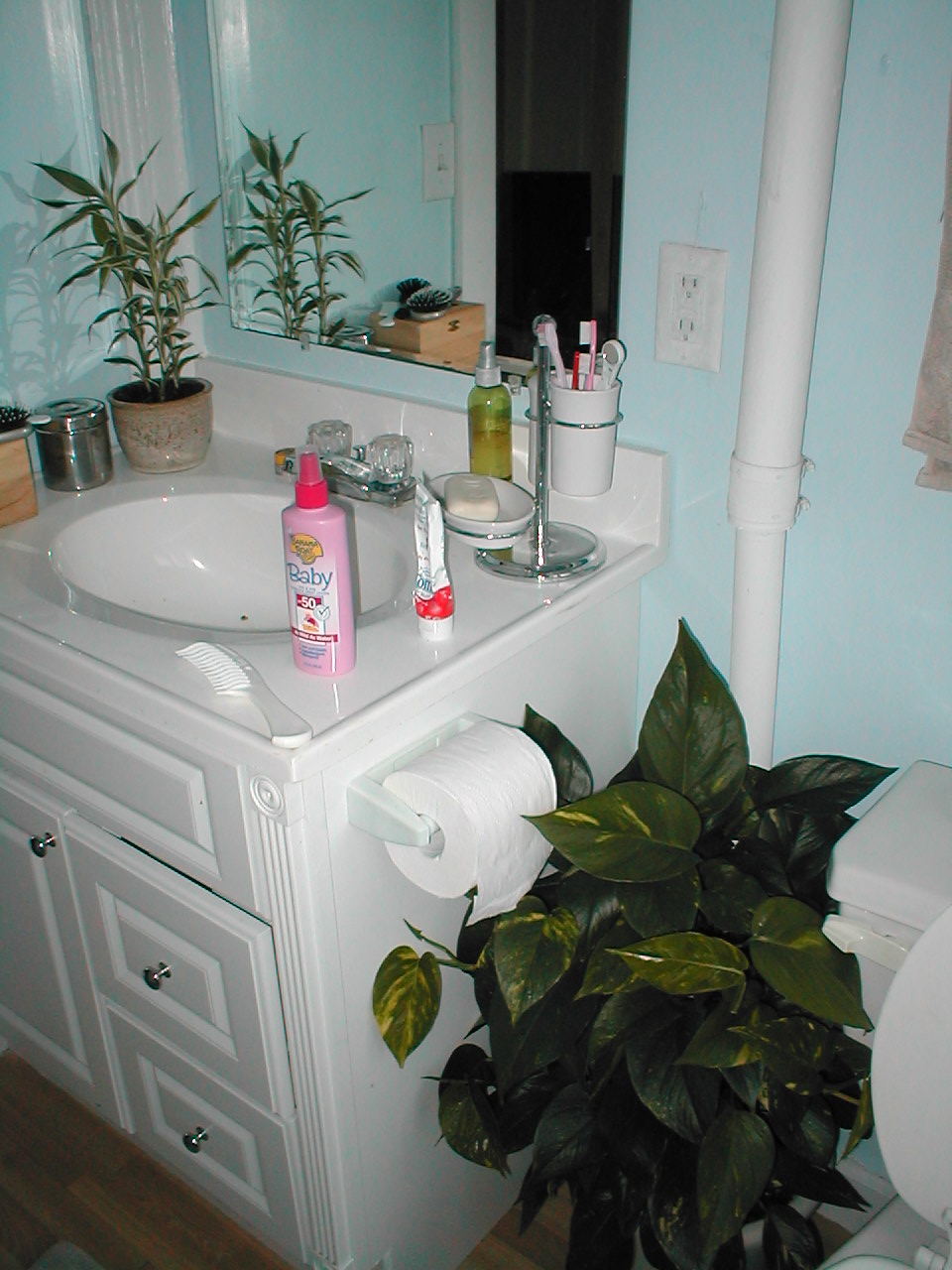The image depicts a bathroom scene viewed through the reflection of a mirror positioned at the top. The room appears dimly lit, with various elements subtly illuminated. In the foreground, there is a white porcelain sink equipped with a silver faucet and crystal-clear handles. To the left side of the sink sits a gray flower vase filled predominantly with green leaves. 

Adjacent to the vase, a sleek silver container is visible. Toward the right, there is a green bottle adorned with a silver cap. On the countertop, there is a white cup holding three toothbrushes—one blue, one red, and one white. A small silver item is placed within the cup. Next to it, a white dish rests on the left side of the sink.

Further to the left on the countertop, a white tube with a red bottom, and a pink bottle featuring a red cap and an image of a baby at the front, are neatly placed. The countertop itself is stark white, matching the overall aesthetic of the bathroom. A white brush and comb lie near the other items. 

Below the countertop, the lower part of the vanity includes white drawers with matching handles. To the right of the scene, an open toilet seat is visible, accompanied by a vertical metallic pole. The soft glow in the image highlights a roll of toilet paper placed near the toilet, while lush green leaves add a touch of nature to the space.